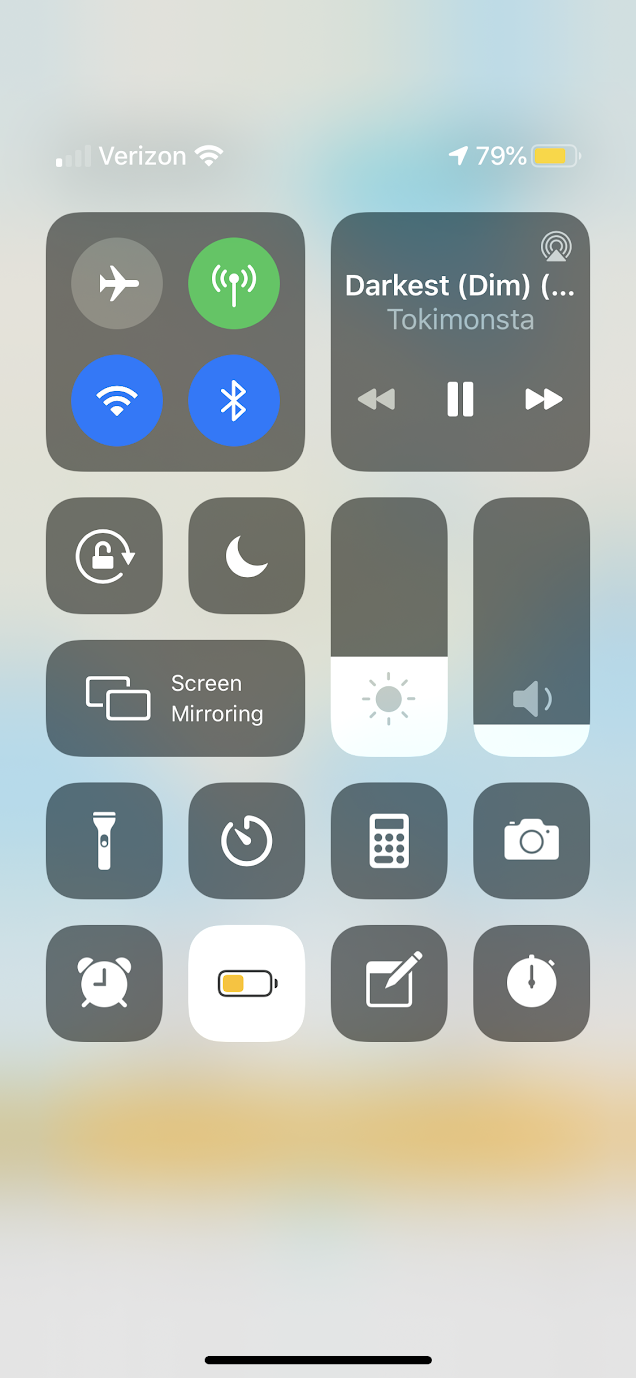This screenshot appears to be from a smartphone or tablet, featuring a light blue background with subtle variations in shades ranging from grayish blue to sky blue. At the very bottom, a very light band of gold adds a touch of warmth. The status bar at the top left displays "Verizon" in white font, along with the Wi-Fi icon represented as an inverted triangle. The battery icon, located on the right side of the status bar, shows a charge level of 79%.

The main portion of the screen is divided into oblong boxes with rounded corners, each containing various icons. In the upper-left corner, icons for Airplane Mode, Bluetooth, and Wi-Fi are visible. To the right of these, a gray oblong shape displays the text "Darkest (dim)" which likely indicates the title of a song currently playing. Below this, the name "Toki Monsta" suggests the artist. Additionally, various icons such as those for the alarm clock, battery, and camera are visible at the bottom of the screen.